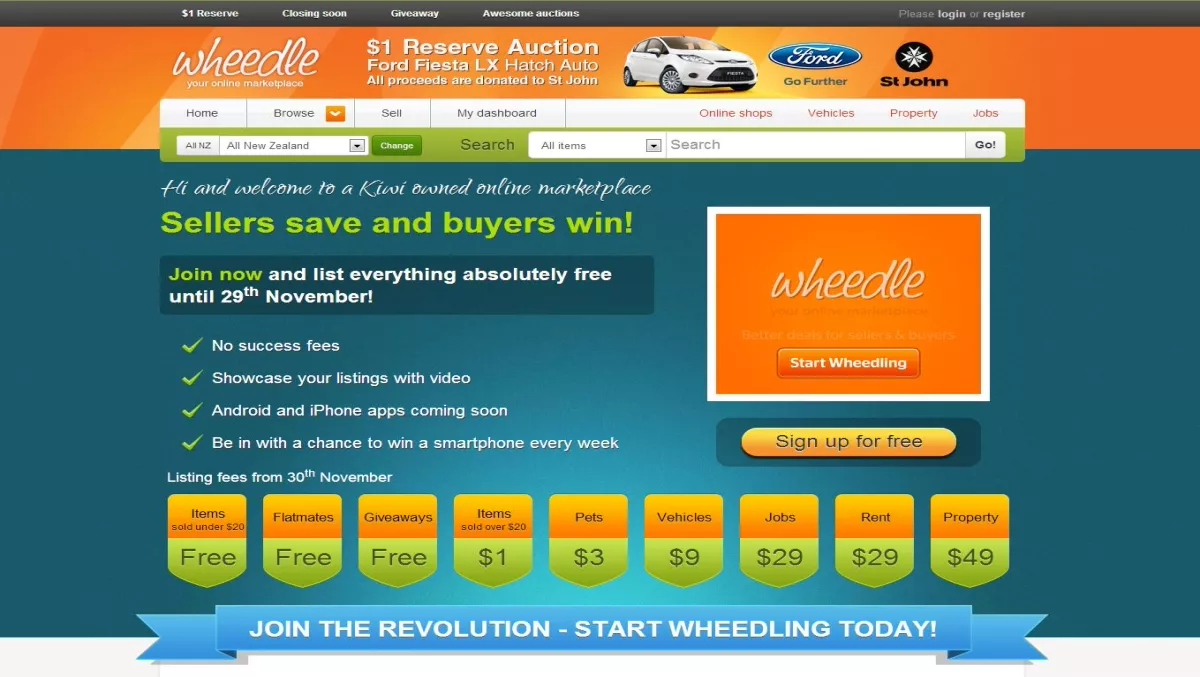**Detailed Description of Image:**

The image appears to be a promotional screen from an online auction site, featuring various elements and textual information as follows:

1. **Header**: The top of the screen has a grey section that prominently displays "One Dollar Reserve" in relation to the site and clothing auctions.

2. **Main Banner**: There is an orange bar with the text "Weedle," indicating the name of the marketplace. Beneath this, it mentions important actions for users, such as logging in and registering.

3. **Auction Details**: The content indicates that the auctions include a variety of items such as suits, a house for auction, and a noticeably highlighted Ford Fiesta car.

4. **Charity Information**: It prominently states that all proceeds from the auctions are donated to St. John's.

5. **Website Navigation**: Links like "home," "browse," "sell," and "bash" are mentioned, suggesting easy navigation to different sections of the site.

6. **Auction Process**: There’s an emphasis on items with a one-dollar reserve, cars including brands like Ford and Honda, and various items listed with categories:
   - Items under $20
   - Giveaway sections
   - Special listings for pets, vehicles, jobs, rentals, and properties with specific listing fees.

7. **User Interaction**: The platform supports actions like "Donate now” and a note that users can list items absolutely free until the marketplace becomes more established. 

8. **Visual Elements**: The image includes check marks indicating features or incentives like showcase videos, upcoming Android app, and a chance to win something listed as "BN."

9. **Marketing Slogan**: It prominently displays the slogan "Join the revolution and start wheeling today!"

10. **Background and Other Elements**:
    - The background is a shade of blue.
    - There is some sort of ribbon present which might signify awards or highlights.
    - Shadows are also mentioned, likely adding depth to the layout.

11. **Footer Information**: It details various categories and costs for listing:
   - Free listings for items under $20.
   - $3 for pets.
   - $10 for vehicles.
   - $29 for jobs and rentals.
   - $49 for property listings.

**Summary**: The visuals strongly encourage user participation in a versatile auction environment, promoting a new marketplace experience with charitable benefits and broad category listings.